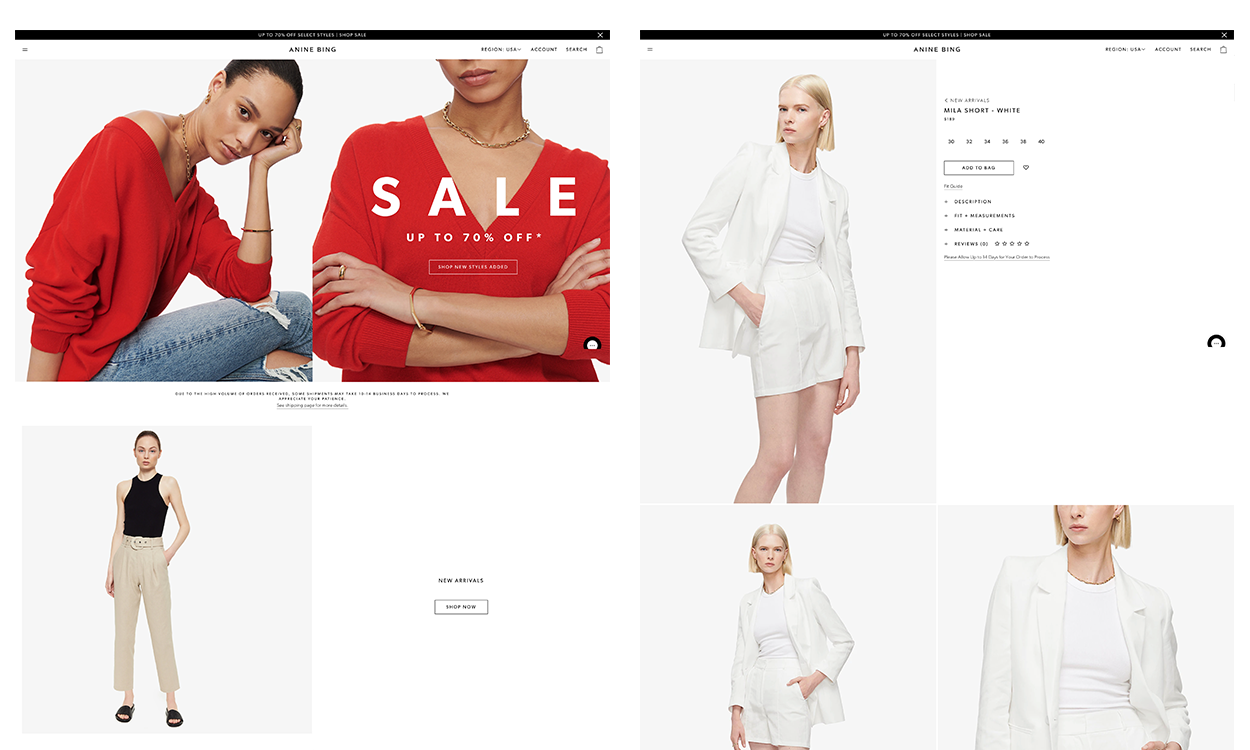The image is a split-panel composition showcasing a clothing store's sale. 

**Left Panel:**
- **Upper section:** A woman with a tan skin tone is showcasing a stylish red blouse with long sleeves and blue pants featuring ripped portions around the knees. She is accessorized with a gold necklace. Positioned at the top right corner of this section is a "SALE up to 70% off" announcement in bold white text.
- **Lower section:** Another woman, looking directly at the camera, is wearing a black tank top, light brown pants, and black sandals. Her hair is cut short.

**Right Panel:**
- **Upper section (larger photo):** The same woman appears, now showcasing almost her entire body up to the calves. She is fair-skinned with blonde hair, and she is dressed in a chic ensemble consisting of a white shirt, a white jacket, and a white skirt.
- **Lower section (two smaller photos):** The woman strikes different poses. In one, she is facing toward her side, and in the other, she is facing the opposite side, providing varied views of her outfit.

Overall, the images collectively highlight diverse clothing options available in the store, complementing the vibrant sale promotion.